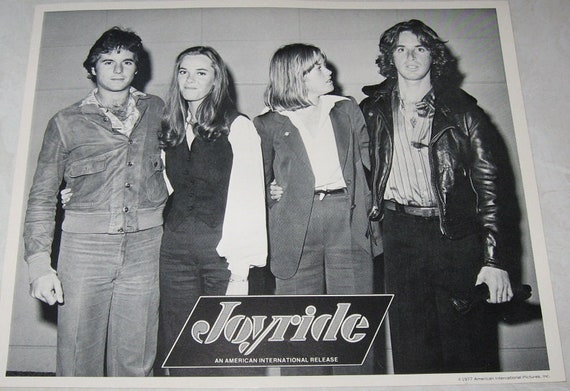The black-and-white photograph titled "Joyride: An American International Release" captures what is likely a band or group from the late 1960s or early 1970s. The photo, which appears to be an album cover, features four members arranged from left to right, each showcasing distinct fashion from the era. On the far left, a man with brown hair and wide 70s lapels stands wearing a members-only style jacket and pants, his arm around a woman next to him. She has long hair flowing past her shoulders and is dressed in a flowing sleeve blouse with a vest and pants ensemble. Next to her, another woman with a bowl cut and shoulder-length hair gazes up to her left at the man beside her. She is attired in a jacket, pants, and a white V-collar shirt. The man on the far right sports long flowing brown hair, a leather motorcycle jacket, a striped shirt, and belted pants, and is holding an object that resembles a flashlight. The photograph angle hints at it being a picture of a picture, suggesting a vintage or retro print style. The composition, logo, and fashion distinctly echo the 70s vibe, presenting a sense of era-specific joy and style.